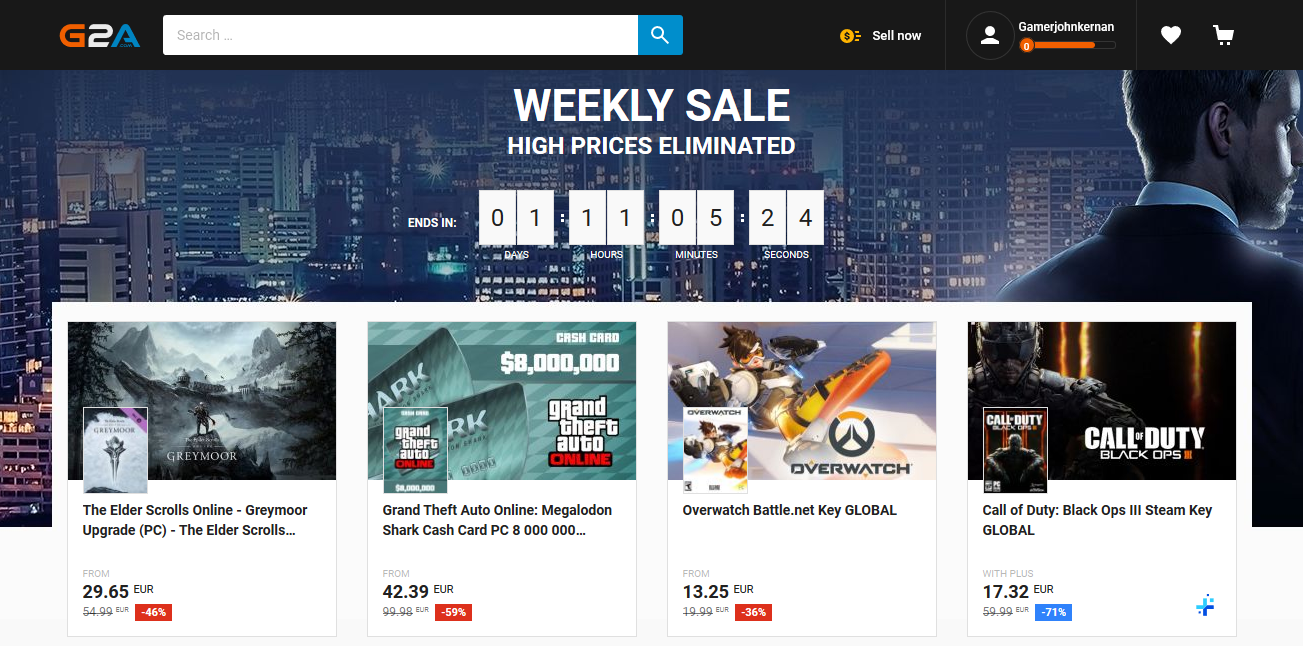**Description:**

The image captures a detailed screenshot of the G2A website homepage. Here's a meticulously formulated description:

---

At the top of the screenshot, a black navigation bar prominently features the G2A logo. The "G" is colored orange, the "2" in white, and the "A" in blue. Following the logo, there is a blue and white search box labeled "Search," with a blue button displaying a white magnifying glass icon. Adjacent to the search box is a gold coin icon next to the text "Sell Now" in white. Additionally, a white icon resembling a head and shoulders cartoon figure represents the user profile, identified by the username "Gamer John Kerman."

Below this section, an orange bar displays icons including a white heart and a white shopping cart. The main body of the website features a nighttime city skyline image, showcasing various buildings illuminated in tan, black, and gray hues. 

To the right of this skyline image is a man with short hair and a beard, dressed in a black suit jacket and white collared shirt. Accompanying this image, text in white promotes a "Weekly Sale - High Prices Eliminated," with a countdown timer indicating "Ends in 1 day, 11 hours, 5 minutes, and 24 seconds."

Below this promotional section, several product listings are displayed:

1. **The Elder Scrolls Online: Greymoor Upgrade (PC)** 
   - Price: €29.65
   - Regular Price: €54.99
   - Discount: 46% off
   - Image Description: A character standing in a desolate, mountainous area under a gray sky.

2. **Grand Theft Auto Online: Megalodon Shark Cash Card (PC)**
   - Price: €42.39
   - Regular Price: €99.98
   - Discount: 59% off
   - Image Description: Contains light blue and tealish graphics.

3. **Overwatch Battle.net Key (Global)**
   - Price: €13.25
   - Regular Price: €19.99
   - Discount: 36% off
   - Image Description: A superhero character with short brown hair in a black and white suit, resembling Iron Man, with an orange leg. The product title "Overwatch" is also visible.

4. **Call of Duty: Black Ops 3 Steam Key (Global)**
   - Price: €17.32
   - Regular Price: €59.99
   - Discount: 71% off
   - Image Description: A figure in black armor, with the title "Call of Duty: Black Ops."

Adjacent to this last product listing, there is a blue plus sign icon.